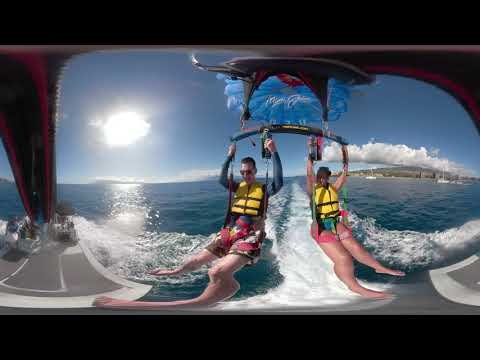The image captures a vibrant scene of two people engaging in parasailing. The man on the left and the woman on the right are both wearing bright yellow life jackets and colorful swimsuits— the man in reddish and greenish swim trunks, and the woman in pink bottoms. They are holding on to a curved black bar that is attached to the parasail, which has a blue balloon inscribed with "Maui Gym" in the background. Both individuals are suspended above the ocean, with their legs dangling near the water, slightly blurred due to motion. The scene is bathed in sunlight, with a clear blue sky and a few scattered white clouds. An island is visible in the background, dotted with sailboats, adding to the picturesque setting.